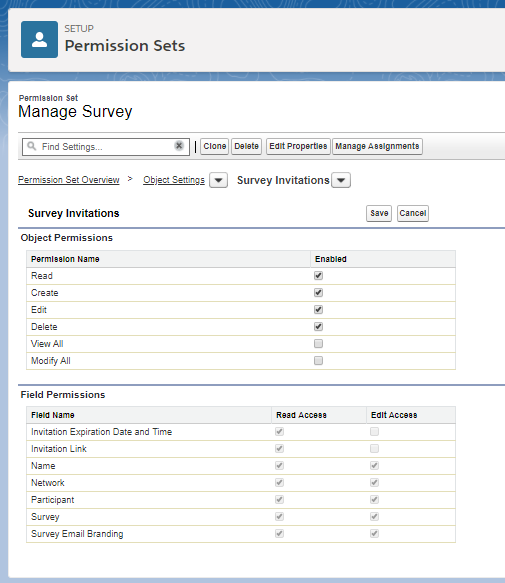The image showcases a comprehensive interface for managing survey permissions and settings. At the top of the page, a text header indicates the section dedicated to "Permission Sets." Below it, various tabs and fields are available for configuring different aspects of a survey.

1. **Setup Section**: This includes various options for managing the survey.
2. **Permission Sets**: Sub-sections such as "Manage Survey," "Find Sets in Search Field" provide functionalities to clone, delete, edit properties, and manage assignments related to the survey.
3. **Survey Invitations**: Includes fields for "Object Permissions," "Permission Name," and toggles for enabling or disabling read, create, edit, and delete permissions.
4. **Checked Permissions**: Indicators for "View All" and "Modify All," showing which settings are checked or unchecked.
5. **Field Permissions**: Detailed fields such as "Field Invitation," "Expression," "Date and Time," "Invitation Link," "Name," "Network," "Participant," and "Survey Email."
6. **Branding**: An option or section to manage branding aspects, likely pertaining to survey emails and participant views.
7. **Permissions Summary**: A summary indicating that all permissions are checked for read and edit access, barring the first two fields—"Invitation," "Expression," "Date and Time," and "Invitation Link," which have specific permissions set.

Overall, the image is a detailed representation of the permission settings and management tools available for a survey, allowing for granular control over read, edit, create, and delete actions.